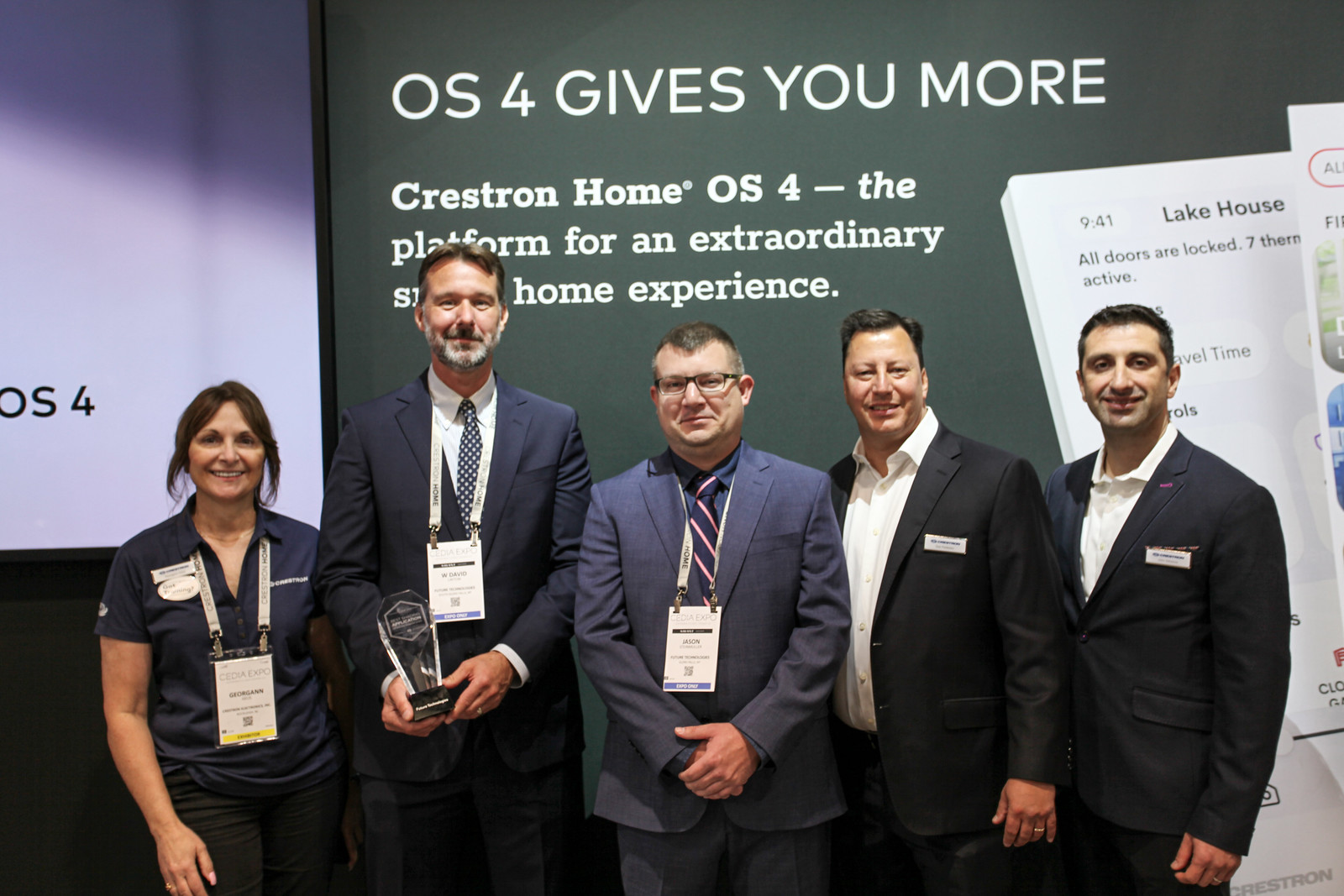In the image, five individuals are standing and posing for the picture against the backdrop of a large billboard. The group consists of a woman on the left wearing a blue polo shirt and four men, two of whom are sporting lanyards and the other two lapel pins. The man standing directly to the right of the woman is holding a small trophy made of glass or plastic with a black base, possibly indicating they have won an award. The men are dressed in dark suits with white shirts, and two of them are wearing ties, while the woman complements their attire with black pants. All five individuals are smiling.

The billboard behind them prominently displays the text, "OS4 gives you more, Crestron Home OS4, the platform for an extraordinary safe home experience." Additionally, there are images of papers or documents on the right side of the billboard. The scene suggests that the group is at an event or summit related to Crestron Home OS4, possibly promoting a sophisticated home automation system.